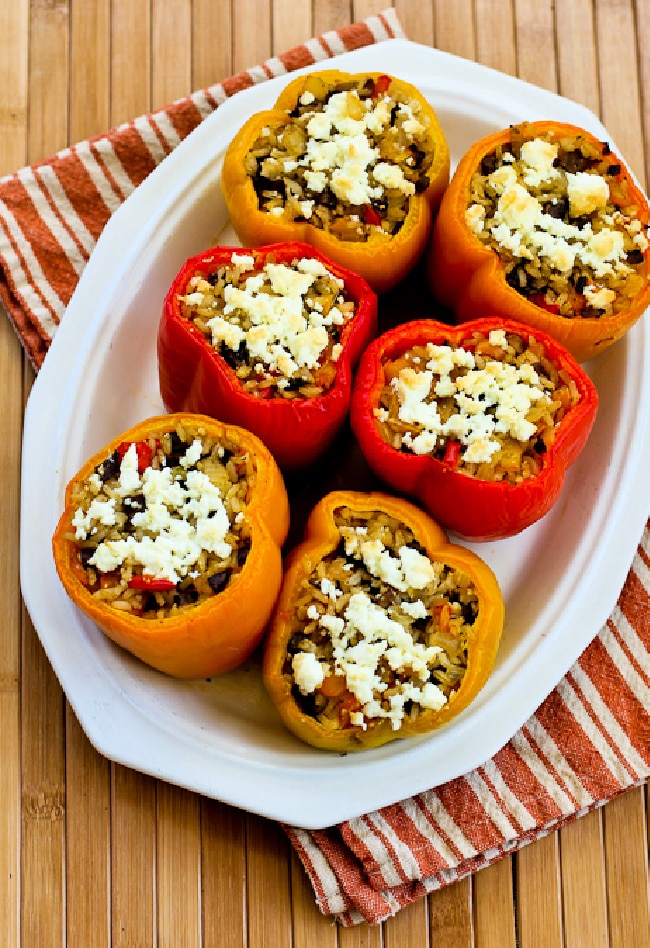The image features six colorful stuffed bell peppers, meticulously arranged on a rectangular oval-shaped white baking dish. The dish is set on a vibrant red and white striped towel, which in turn rests on a wooden table, adding a rustic charm to the scene. There are four orange peppers and two red peppers, aligning in a pattern with two orange at the top, two red in the middle, and two more orange at the bottom. Each pepper is halved and generously filled with a hearty mixture that appears to include rice, beans, and finely chopped bits of pepper. The stuffing is crowned with a layer of white cheese, potentially feta, adding a tasty finishing touch. The presentation suggests the dish is either ready for baking or freshly baked, enhancing its mouth-watering appeal.